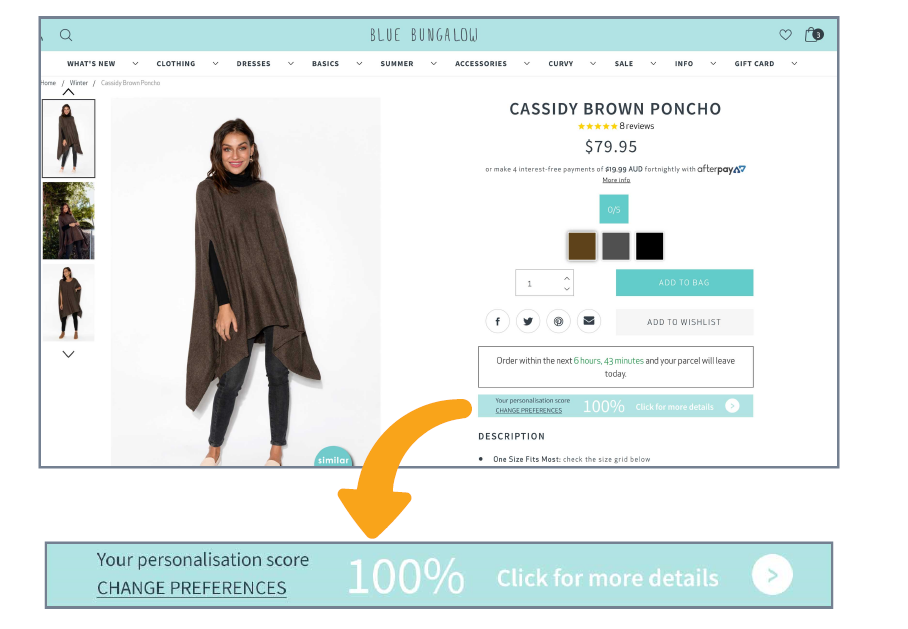The image features a fashion website with an aqua greenish banner displaying the text "Blue Bungalow" at the top. On the left side of the banner, there is a magnifying glass icon indicating a search function. Opposite, on the right side, there is a heart icon inside a shopping bag with a circled number "3," which is blue with a white numeral, signifying three items in the cart.

The website's menu is located on the left-hand side and includes categories such as "What's New," "Clothing," "Dresses," "Basics," "Summer," "Accessories," "Curvy," "Sale," "Info," and "Gift Card," each with drop-down arrows for further navigation.

Adjacent to the main content area, there are three small thumbnail images next to a larger primary image. The primary image showcases a woman with a tan complexion, long brown hair, and a beaming smile. She is wearing a long pull-over garment resembling a poncho, paired with skinny jeans. The text beneath the image reads "Cassidy Brown Poncho," accompanied by a 5-star review rating and a price of $79.95. Four color options are displayed in small boxes beneath the description.

Additionally, there is a box next to this section with the numeral "1," social media links, and another box featuring an orange arrow pointed downward labeled "100%." A "Click more for details" prompt appears beside it, accompanied by a clickable circle with an arrow inside.